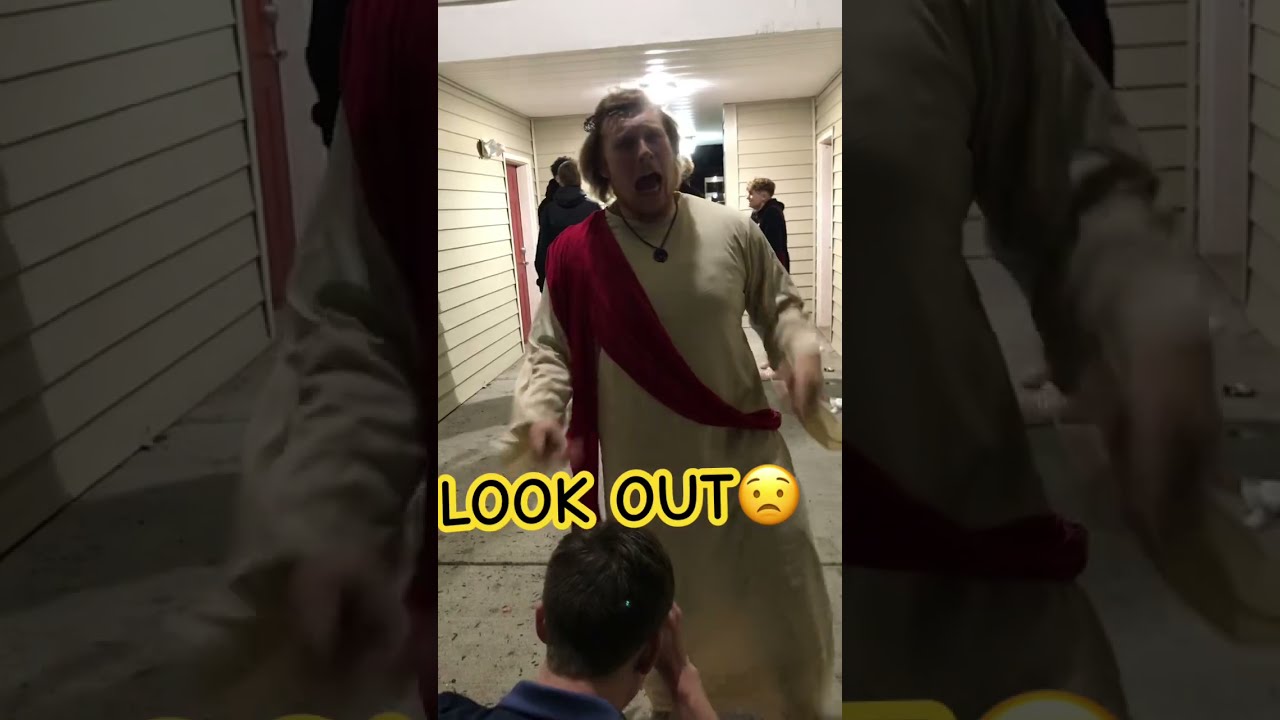In this night-time photograph, likely taken on a cell phone and resembling a scene from a TikTok video, a man evocatively dressed as Jesus stands at the focal point. Clad in a white robe with a red sash, the man, who appears to be of Caucasian descent, has messy brown hair and is wearing a black necklace with a pendant. His eyes are closed, his mouth is wide open, and his arms are extended in a dramatic, possibly screaming gesture. Kneeling in front of him, with his back to the camera, is another man with short brown hair, dressed in a blue-collared shirt, seemingly taking a photograph. 

In front of the robed man, the text "Look out!" is prominently displayed in yellow outlined, black-lettering, accompanied by a frowning face emoji. The background reveals an interior hallway with beige clapboard walls and a white door to the left. Several figures in black hoodies are standing on the concrete floor, suggesting a social or communal gathering. 

This main image is positioned within a centrally aligned, vertical rectangular box. Darkened, enlarged fragments of the same image frame either side, adding a surreal, layered effect to the scene, making the robed man’s extended arms particularly prominent on the left and right thirds of the frame.